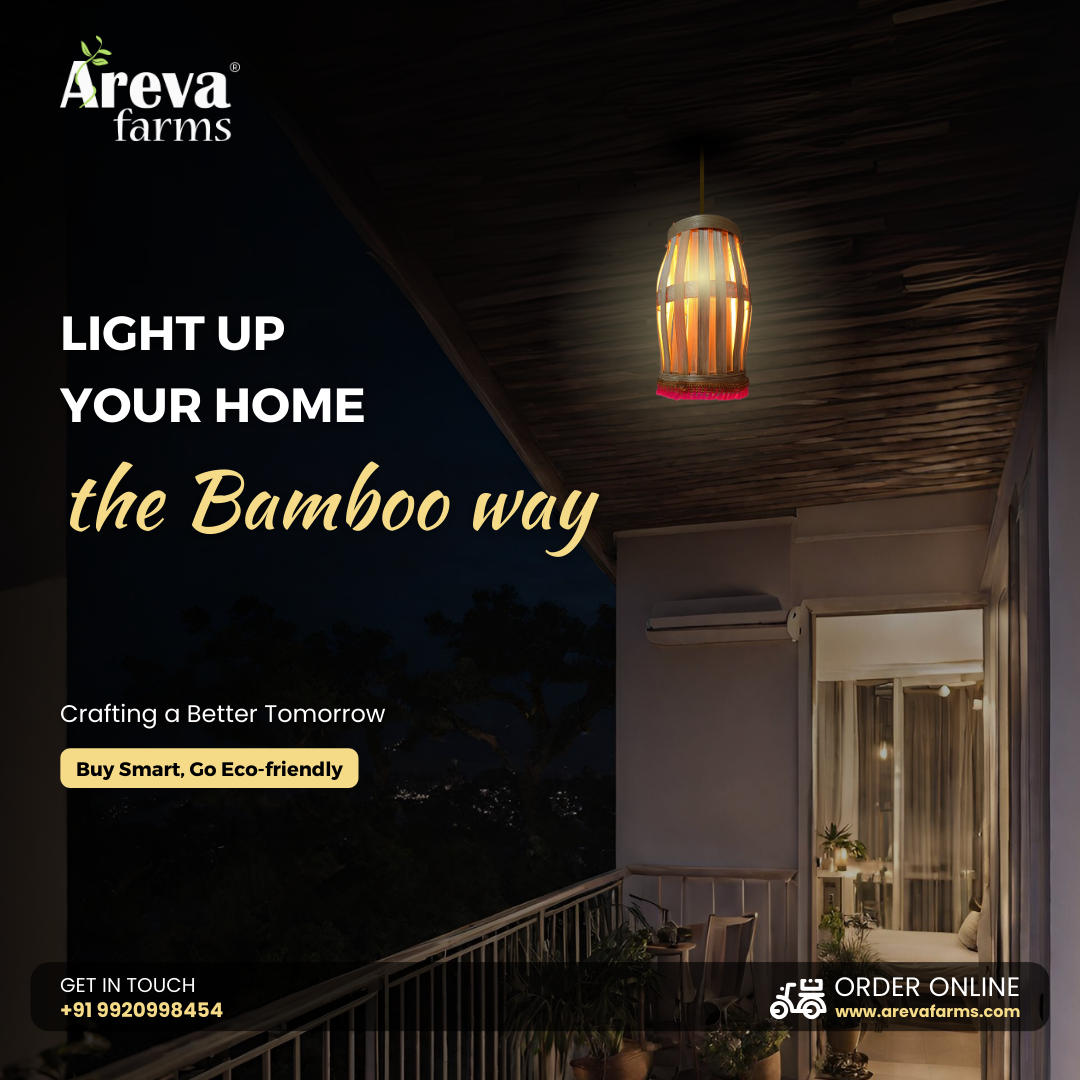The advertisement for Arvia Farms prominently features their eco-friendly bamboo lamps. In the upper left, the company logo “Arvia Farms” is displayed in white font, with a green sprig entwined around the 'A' in 'Arvia'. Below this logo, the tagline "Light up your home the bamboo way" is written, where "Light up your home" is in white sans serif, and "the bamboo way" is in muted yellow script. Further down, the ad emphasizes sustainability with the phrase "Crafting a better tomorrow," followed by a call to action in a muted yellow rounded rectangle that reads, "Buy smart, go eco-friendly."

On the right side of the advert, there is a picturesque image of a house porch lit by a stylish bamboo lamp, which hangs from a wooden roof. The warm light from the lamp illuminates the porch, and you can catch glimpses inside the house through the windows. At the very bottom right, a small graphic of a motorcycle indicates delivery options, along with text that prompts viewers to "Get in touch" followed by a contact number, and encourages online orders at www.arviafarms.com. The comprehensive design and focused messaging underline Arvia Farms’ commitment to sustainable living through their bamboo products.